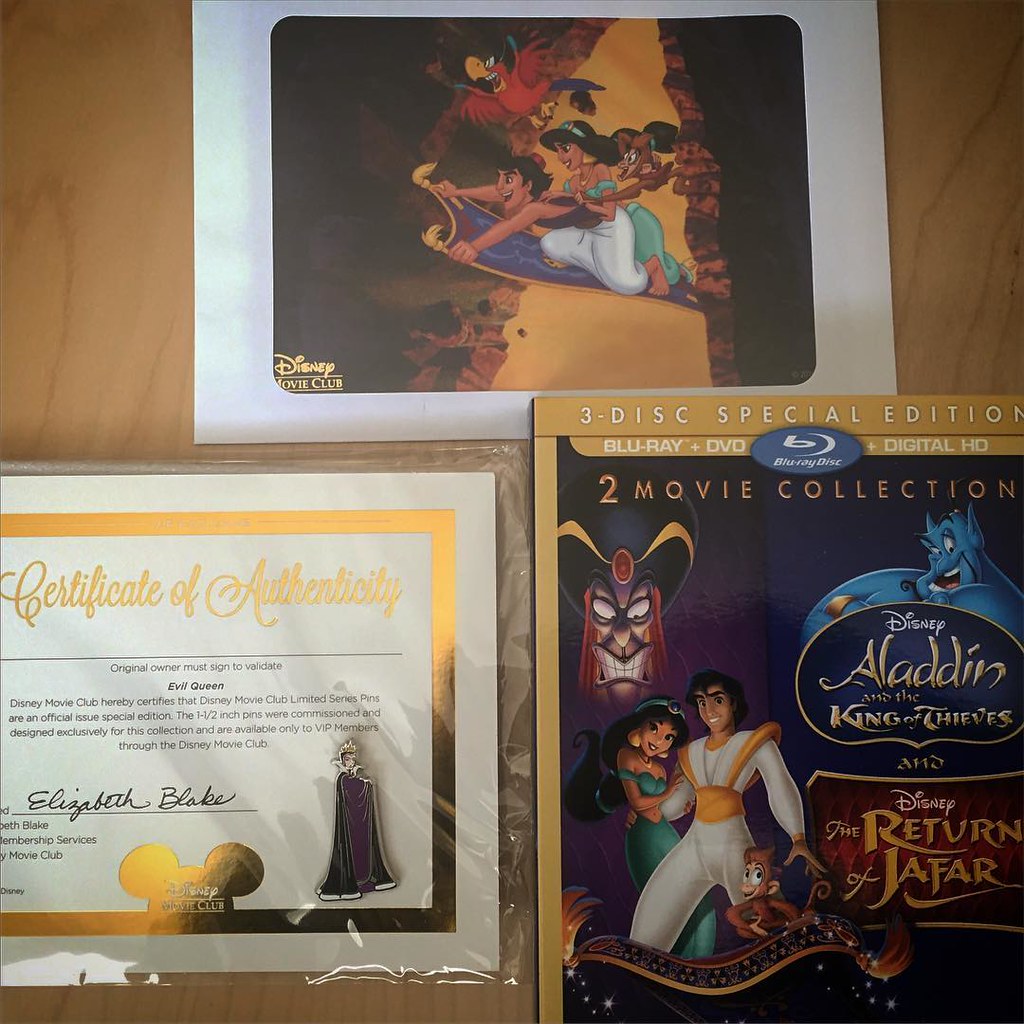The square image showcases a lively Aladdin-themed collection set against a brown tabletop. Dominating the upper middle section, there's a vibrant photo of various cartoon characters who appear to be of Arabic origin. A male character, likely Aladdin, is depicted riding a magic carpet with Princess Jasmine dressed in white beside him. Above them hovers a red parrot, and to the right, a small brown animal—presumably Abu the monkey—adds to the scene.

In the lower-left corner, a certificate of authenticity framed in gold script, addressed to Elizabeth Blake, is prominently displayed. Below this, a gold outline of Mickey Mouse ears subtly symbolizes its Disney origins.

To the right of the certificate, there's a cover for a deluxe edition Blu-ray set, titled "Aladdin: King of Thieves/The Return of Jafar." Aladdin, wearing a white uniform with gold accents, stands prominently on it, with Princess Jasmine to his right and a grinning villain looming above them. This set is labeled as a "Three Disc Special Edition" and "Two Movie Collection" in gold lettering on a dark border, reinforcing its exclusive status.